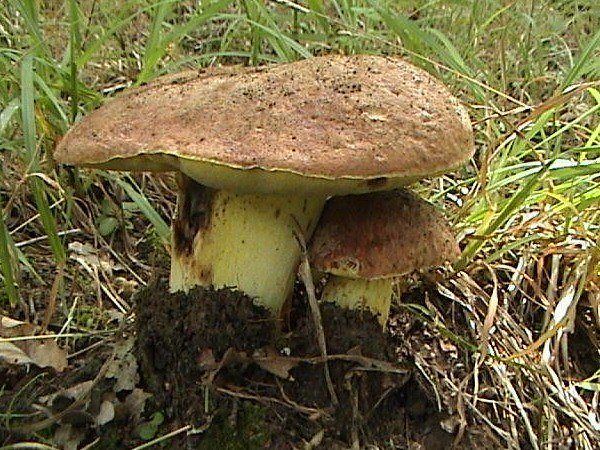The image showcases an outdoor scene featuring two mushrooms emerging from the ground. The larger mushroom, located on the left, has a distinct flat, rounded, medium-brown cap and a pale yellowish stem that appears marked and weathered. In contrast, the smaller mushroom on the right has a similar structured but less prominent brown cap, and its yellowish stem is partially obscured by surrounding dirt and weeds. The mushrooms are nestled in a ground filled with dirt and scattered brown and green weeds, with some additional small mushrooms poking through the dirt on the left. Beyond the immediate foreground, there is an expanse of long, bending grass which appears to have patches with a yellowish tint, possibly illuminated by sunlight. The scene is accentuated with grasses and weeds in varying shades of green and brown, adding to the natural and untamed feel of the environment.